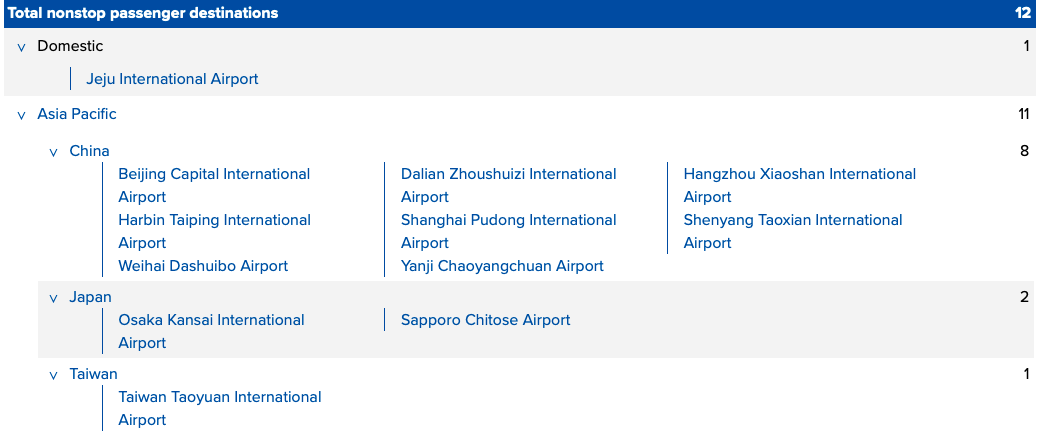This image showcases an informative display divided into three sections representing different regions within the Asia-Pacific category: China, Japan, and Taiwan. The display lists total non-stop passenger destinations, providing detailed information for each region.

The China section includes:
1. Beijing Capital International Airport
2. Shanghai Pudong International Airport
3. Guangzhou Baiyun International Airport
4. Harbin Taiping International Airport 

The Japan section lists:
1. Kansai International Airport

Lastly, the Taiwan section features:
1. Taiwan Taoyuan International Airport

Adjacent to each section, numerical indicators show the count of airports within each category: China with eight, Japan with two, and Taiwan with one. This display emphasizes the numerous direct flight destinations available, facilitating non-stop, one-way travel across these prominent Asian destinations.